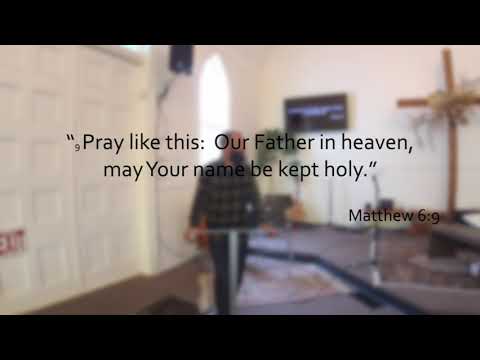In this image, set within a room that appears to be a church, the dominant colors are black, white, and brown, with the top and bottom portions of the image letterboxed in black. The slightly blurred background showcases a bearded man in a dark, checkered flannel shirt and dark-colored pants. He stands at a silver podium, with his hands resting on it, facing us but glancing to his right. The scene includes an off-white wall adorned with a brown wooden cross, possibly decorated with flowers, alongside a mounted TV screen. To the left, there are tall double doors, and an arched window naturally lights the space. The text superimposed over the image, in black letters, reads, "Pray like this, 'Our Father in Heaven, may your name be kept holy,'" and is attributed to Matthew 6:9 from the Bible.